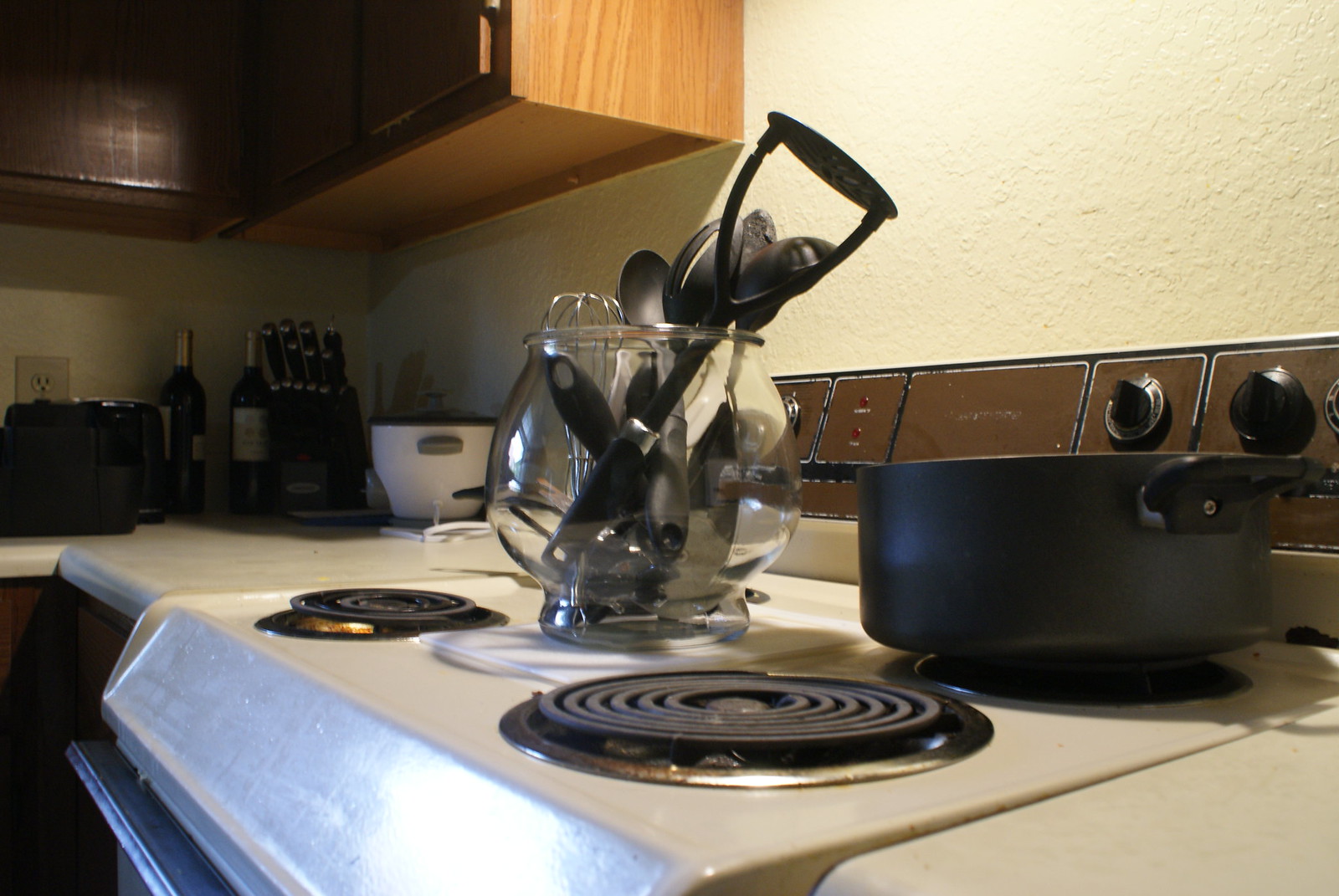A detailed image captured in a home kitchen focuses predominantly on an electric stove with four coil cooking surfaces. The stove features a conspicuous black pot positioned on the back right burner, which appears to be active as suggested by the turned-on knobs located on the stove's rear panel. Centrally placed on the cooking surface is a white cutting board, on which rests a large, transparent glass bowl filled with various cooking utensils. Visible among these utensils are a whisk, serving spoons, and what looks like a potato masher, all protruding above the rim of the bowl due to their considerable size.

The cooking surface and the adjacent countertop share a matching beige hue, though they display signs of wear with slight rust and dirt present. The textured background wall is similarly colored in a beige-cream tone, providing a cohesive look throughout the kitchen. Towards the left of the image, wooden cabinets are visible; these feature a lighter wood grain on the sides and a darker, richer brown on the front panels.

In the background, various kitchen items are neatly arranged, including a knife set, a casserole dish, a crock pot, and two bottles of wine. These additional elements contribute to the warm, functional ambiance of this well-used kitchen space.